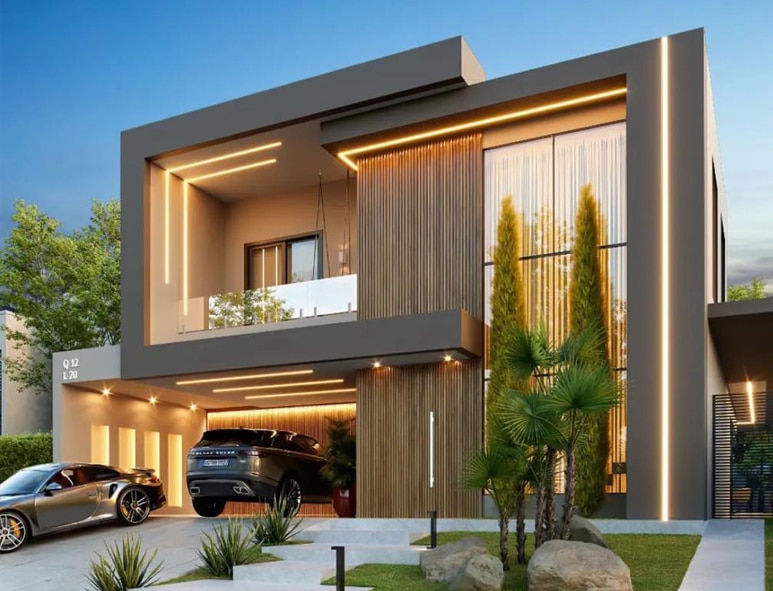The image showcases a highly modern, vividly contemporary house with a striking design combining gray concrete and brown wooden slats, shaped into various interlocking cubes and rectangles. At the forefront is a concrete driveway leading to an open garage, brightly illuminated with yellow and LED lights, revealing a Range Rover parked inside. A metallic silver Porsche is visible in the sloped driveway, bordered by large succulents and small patches of green lawn adorned with big boulders and slender trees, including palm trees.

Above the garage, which is located on the left-center of the structure, the house features an arrangement of tall, vertical and horizontal windows. The second story includes a glass patio with a door, framed by golden-tinted lights. To the right side, a series of large, vertically aligned windows, some with golden curtains, adorn the building. A small gated section and a black bar door are also part of the facade, contributing to the overall striking and geometric aesthetic of the home. The scene is set against a vivid, bright blue sky with additional trees in the background.